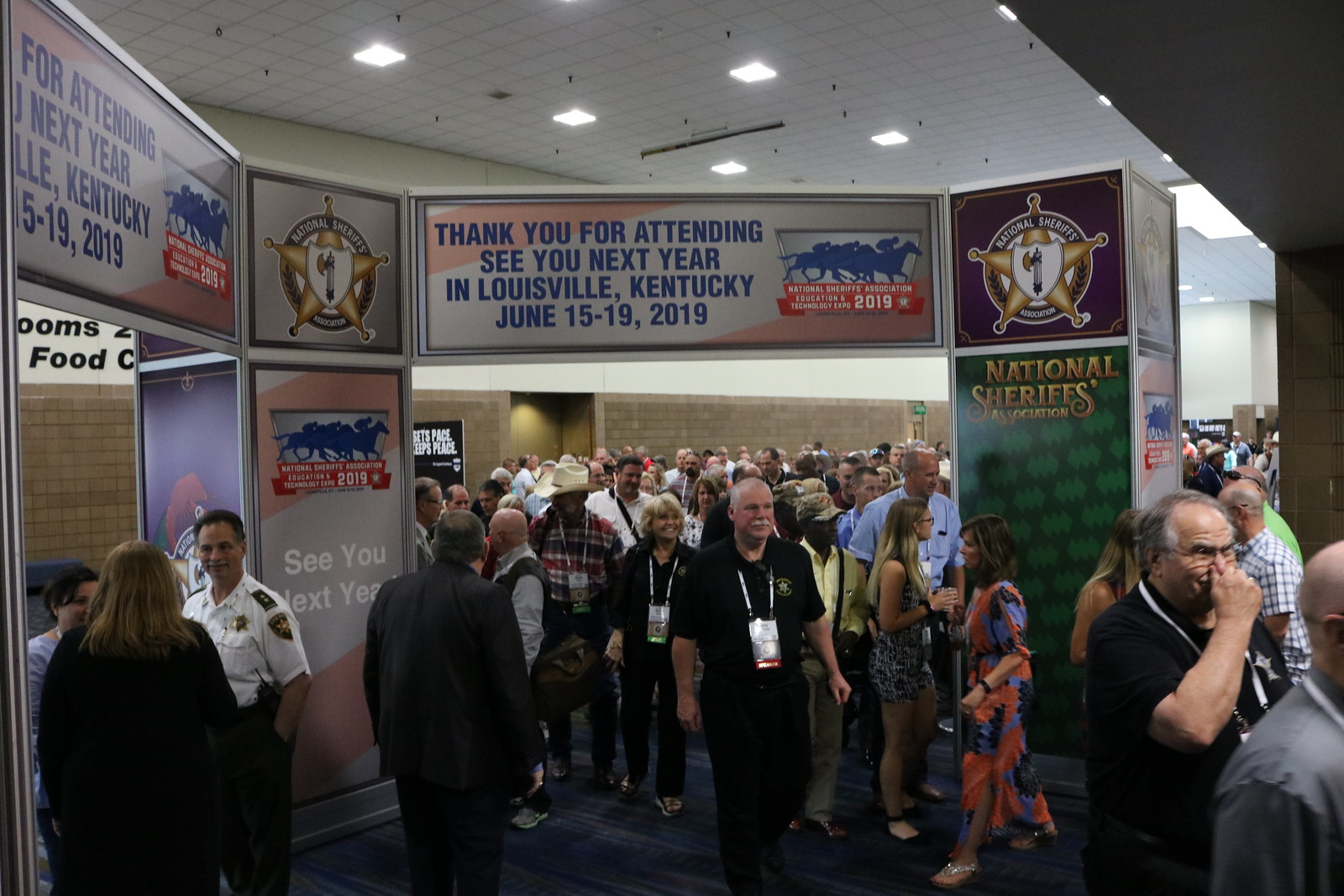The image depicts a bustling scene inside a large room filled with attendees at a National Sheriffs Association meeting. Prominent signage at the top of the image reads, "Thank you for attending. See you next year in Louisville, Kentucky, June 15th to 19th, 2019," in bold, blue capital letters. A logo featuring a gold star with a gray shield that reads "National Sheriffs Association" is also visible. The crowd is diverse and dense, with many individuals wearing lanyards. 

In the center, a bald man with a white mustache stands prominently, flanked by a smiling blonde woman behind him, exhibiting a toothy grin. Behind her, a dark-skinned man is seen wearing a checkered red, white, and black long-sleeved shirt, paired with black pants and a cowboy hat. To the right, another man with silver hair, dressed in a black short-sleeved t-shirt, is holding his hand over his nose. On the left side, a security guard in a white t-shirt is noticeable amidst the large gathering. Cardboard cutouts forming archways and text with blue and gold lettering add to the event's decor, reinforcing the theme and providing additional information about the conference.